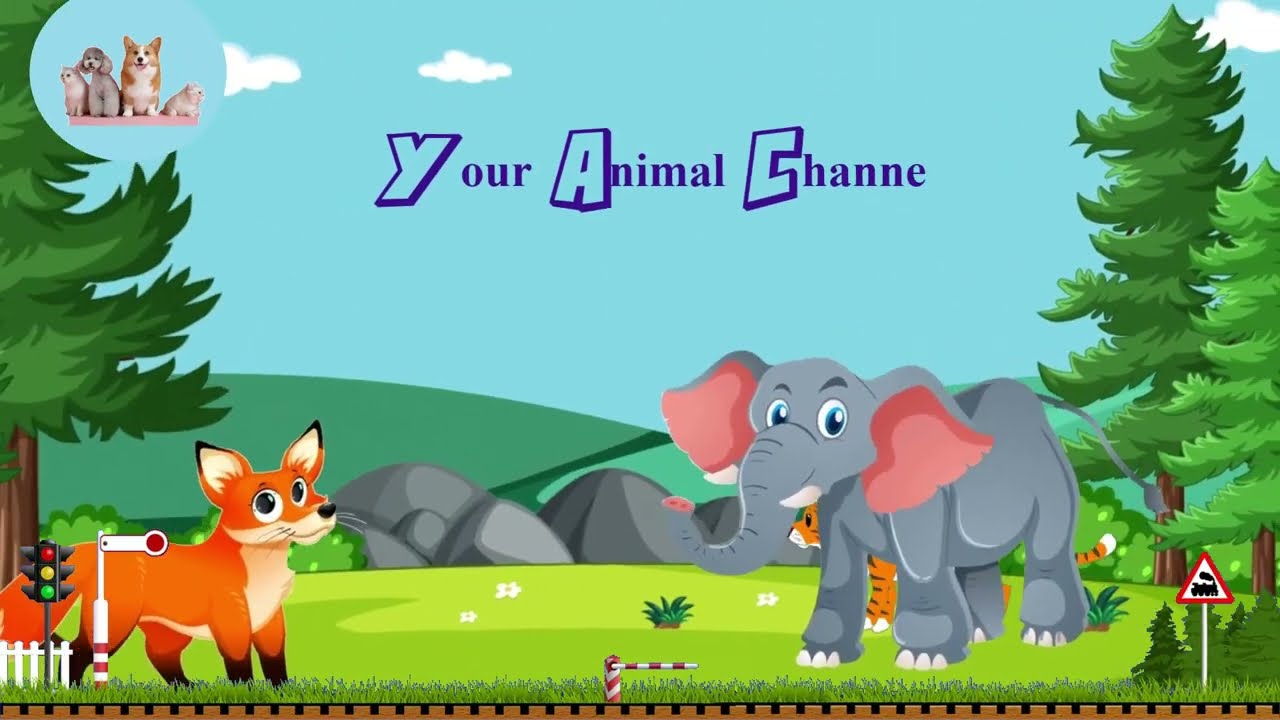The cartoon image depicts a whimsical scene full of vibrant details and various animals against a scenic backdrop. In the lower left corner, there's a cartoon fox standing near a traffic light displaying red, yellow, and green lights and a rail crossing sign. Across to the right, a cartoon elephant stands beside a triangular traffic sign featuring the silhouette of a steam train. Behind the elephant, a tiger peers to the left. At the bottom of the image, a railway line made of brown strips with black dots stretches from the bottom left to the bottom right. The midsection shows a vast field with green grass, colorful flowers, and numerous boulders leading up to a distant mountain range. There are also trees scattered around – two on the right and a large one on the left. Higher up, a bright blue sky with fluffy white clouds sets the tone, and floating in the top left corner is a light blue circle with a pink rectangle containing four animals: a cat, a small grey dog, a corgi, and another cat. At the very top center of the image, blocky blue text reads "Your Animal Chan" with distinctive capital letters. The overall setting gives the impression of a lively and animated forest scene.